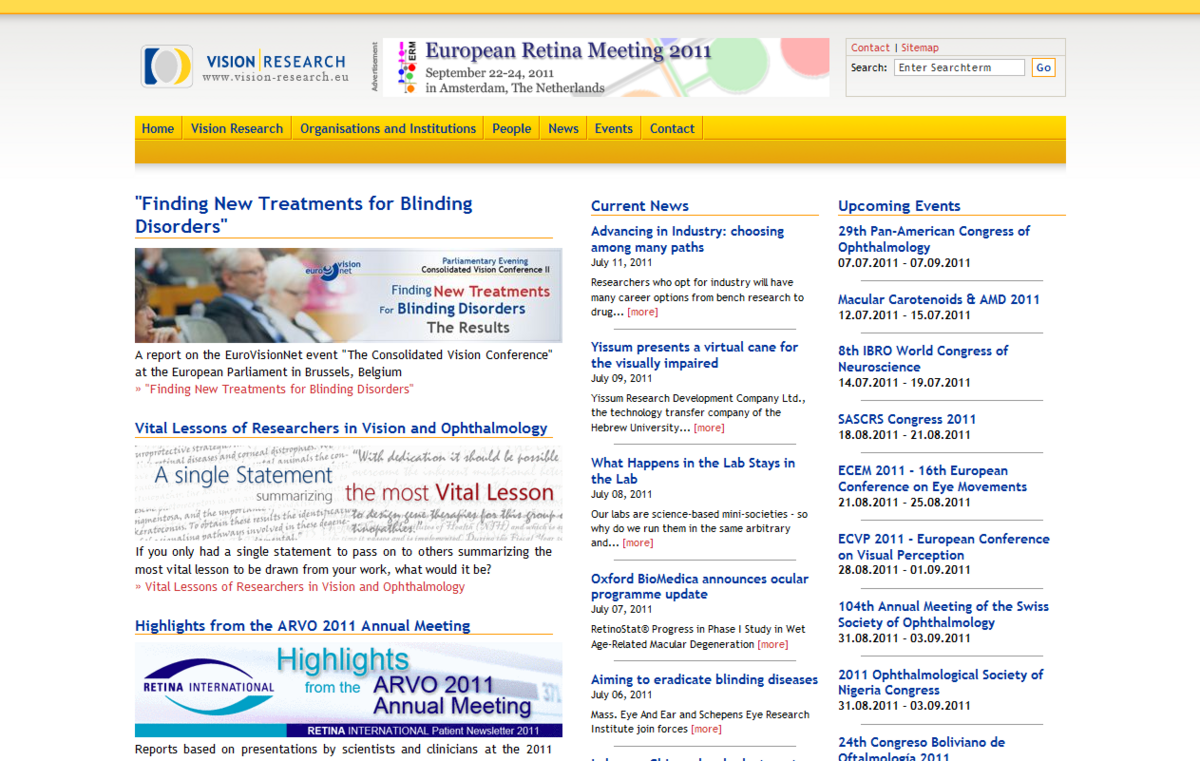The image showcases a webpage for Vision Research, a platform dedicated to addressing eye-related issues. The website URL is prominently displayed: www.visionresearch.eu. The logo features an eyeball, with the left side in blue and the right side in gold. The text "Vision Research" is in blue while the website address is in grey.

To the right of the logo, an announcement for the European Retina Meeting held in September 2011 in Amsterdam, Netherlands, is visible, accompanied by several logos. The site includes a search bar for easy navigation.

A broad, two-toned gold bar sits beneath the header, with menu options such as Home, Vision Research, Organizations, Institutions, People, News, Events, and Contacts, plus room for additional tabs.

Below the menu, there's an article titled "Finding New Treatments for Blinding Disorders," linked for further reading. It mentions a report on the EuroVisionNet Event, highlighting key takeaways from researchers in vision and ophthalmology. It poses the question: "If you only had a single statement to pass on to others, summarizing the most vital lesson drawn from your work, what would it be?" The article seems to include insights from various researchers.

Additionally, the content references highlights from the AeroVo 2011 meeting, noting its relevance for professionals treating or researching blindness. Overall, the website serves as a valuable resource offering access to conferences and scholarly articles for those working in vision research and ophthalmology.